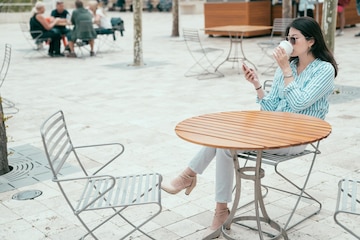In this detailed photograph, a stylish woman is seated in an open-air public courtyard adorned with white stone and tiled flooring. She occupies a white, wireframe patio chair at a circular table with a medium-shiny wooden tabletop supported by a steel base. Dressed impeccably in white pants, beige high heels, and a long-sleeve blue and white striped shirt, she exudes modern elegance with her long black hair cascading over her shoulders, and aviator sunglasses shielding her eyes. Her posture is relaxed with her legs crossed as she looks intently at her cell phone in one hand and holds a white coffee container with the other hand. The serene ambiance of the courtyard is punctuated by additional seating arrangements, including several empty chairs around her table. In the background, particularly in the upper left corner, a group of four people, casually dressed in tank tops, shorts, and long hair, are seated together, adding a lively contrast to the scene. The entire setting, reminiscent of an open-roof café, combines style, serenity, and social vibrancy.